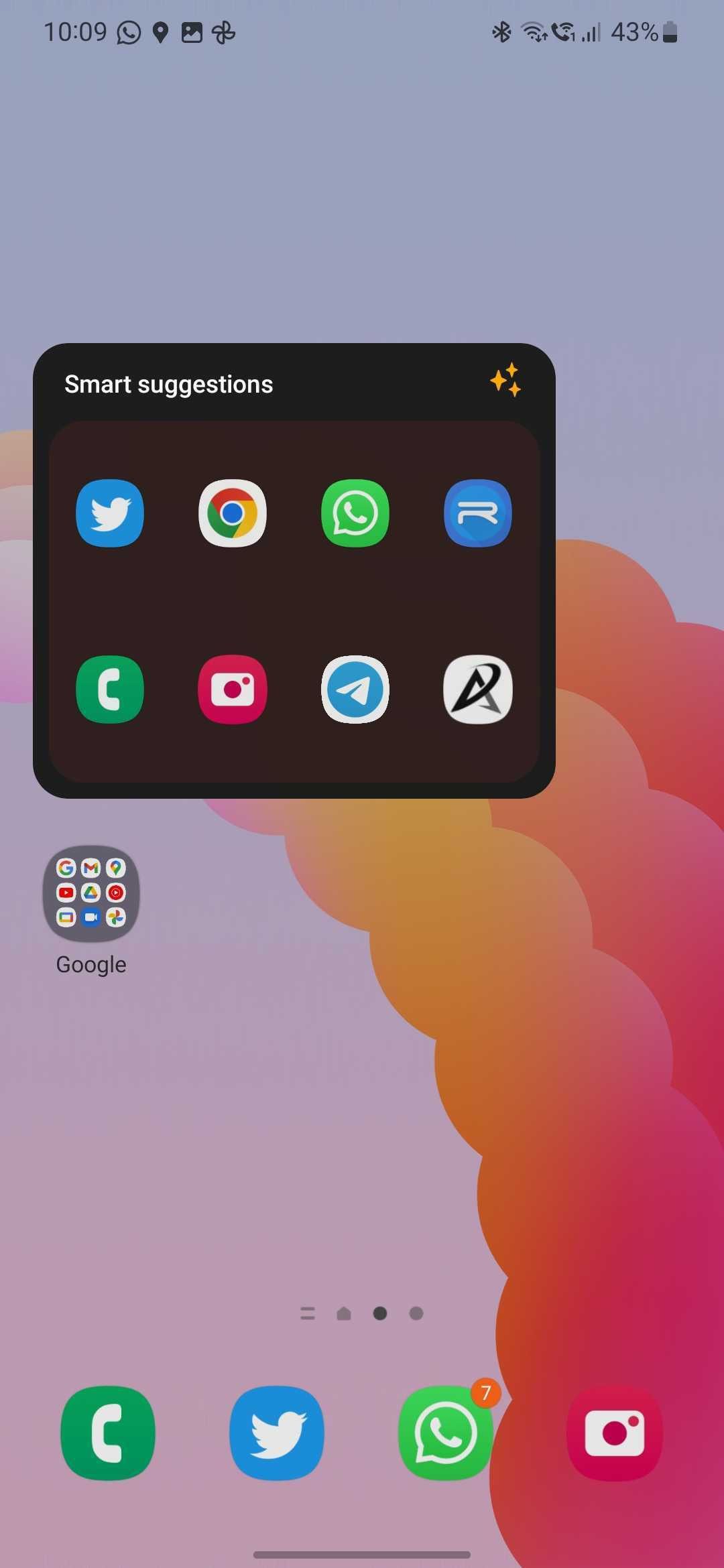The image depicts the screen of a smartphone. The current time is 10:09, indicated in the top left corner next to a notification badge. Directly to the right are several icons, including a photo symbol and others which are not easily identifiable. On the top right corner, the battery is shown at 43% with the icon displaying it below half. There are also icons for Bluetooth and cellular signal strength, which shows three out of the maximum bars, indicating a good connection.

Dominating the center of the screen is a section labeled "Smart Suggestions," showing eight app icons. These include familiar apps such as Twitter, a messaging app, a photo app, a phone app, and an app with a paper airplane commonly associated with messaging or social media.

Below this section is a smaller square containing nine more app icons, unlabeled and too small to identify. Underneath this square, there is a Google search bar.

At the very bottom of the screen are four navigation dots, suggesting multiple home screens. Additionally, there is a dock with four essential apps: a phone app represented by a green circle, the Twitter app, a green messaging app, and a camera app.